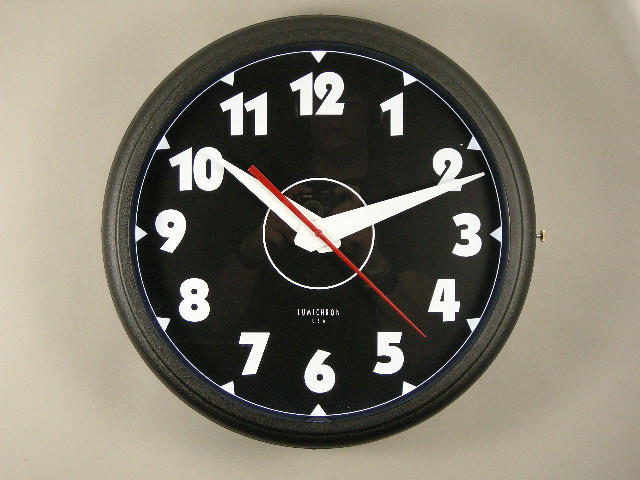In this landscape-oriented photograph, there is a circular clock prominently displayed. The clock features a black frame that appears to be made of plastic, encasing a matching black face. Adorning the face, the numbers 1 through 12 are depicted in bold, white bubble text, arranged in a clockwise direction. Above each numeral, a small white triangle serves as an additional marker. 

The clock's hour and minute hands are white and pointed, contrasting sharply against the dark background. Overlaying these is a slender, red second hand. The time indicated by the clock is 10:12. Beneath the center where the clock hands pivot, there are some white letters, although the text is not legible. The clock is mounted on a wall painted a medium gray, serving as a neutral backdrop that highlights the clock's features.